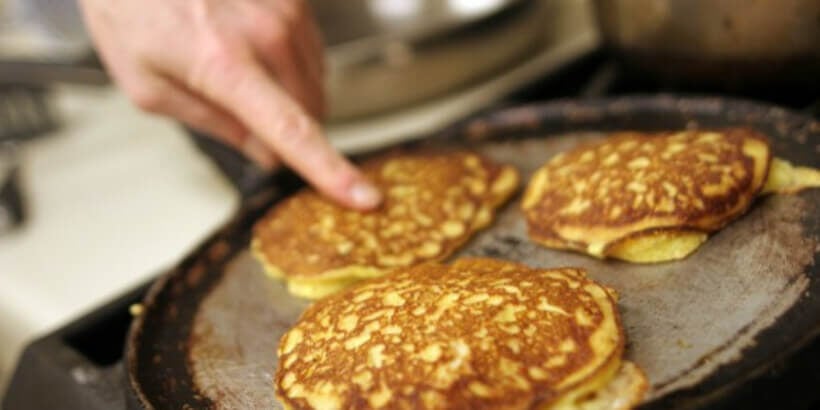The close-up photograph features a well-worn metal pan in the bottom right-hand corner, partially in focus amid a predominantly blurry background. Within the pan, which has a short, sloping upper ridge and a dull gray interior, three equally spaced pancakes are cooking. A human finger with pale skin is seen touching one of the pancakes, extending from the top edge near the left side of the image. The pan appears heavily weathered and sits on what might be a hot plate or stove. In the background, a silver pan is visible, though it is quite blurry, emphasizing the detailed focus on the pancakes and the interacting hand.